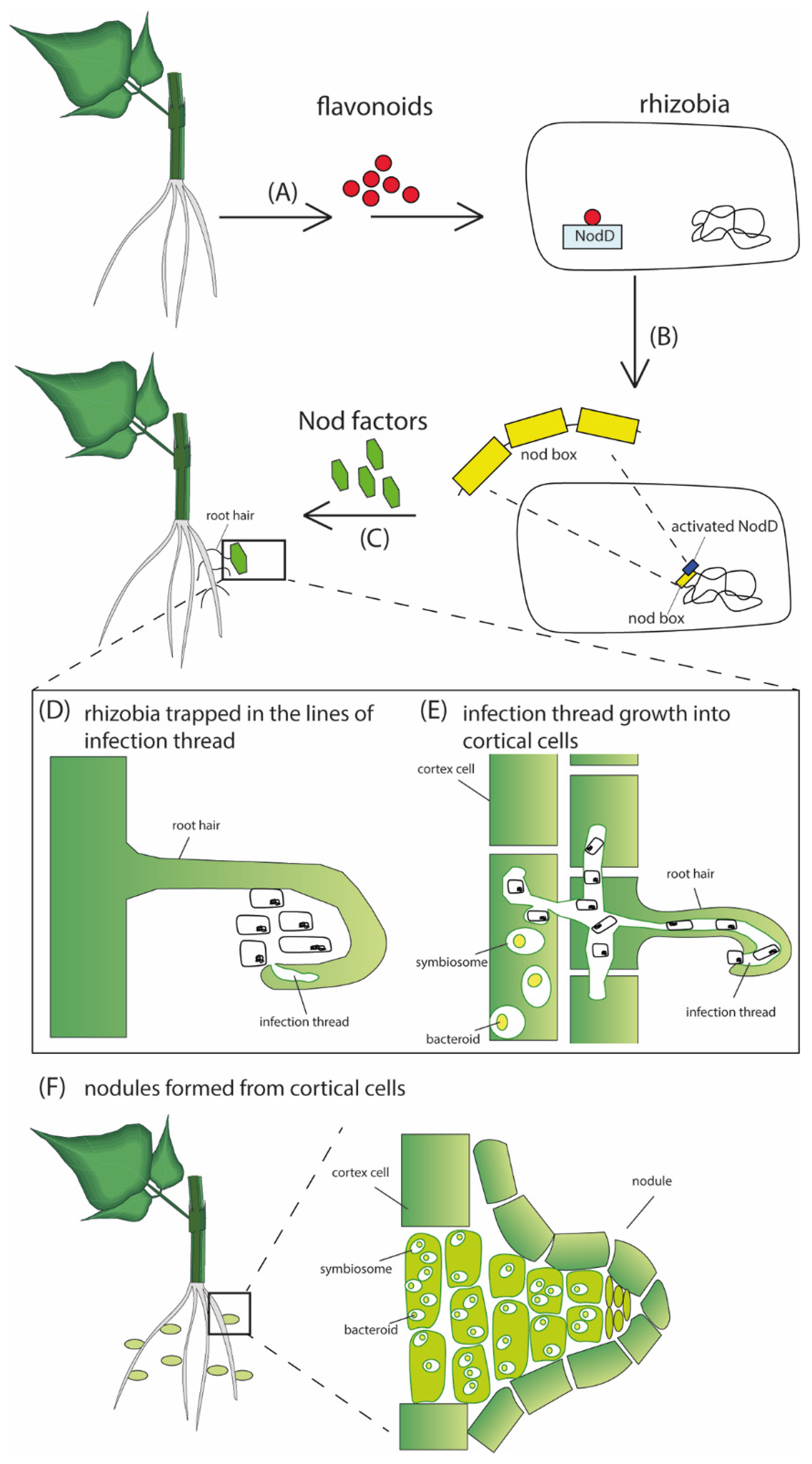This scientific flowchart illustrates the formation of nodules from cortical cells in plants. Starting at the top left, the diagram depicts a plant with a stem carrying three leaves and roots hanging below. The process begins with red-dotted flavonoids (A) moving towards rhizobia, indicated by an arrow. These flavonoids activate the "nodule box," denoted by another arrow (B). The action continues as arrow C guides the activated elements back to the left into the root hairs, enlarging the image below. At point D, rhizobia are trapped in the lines of an infection thread within the root hair. Following this, arrow E shows the infection thread's growth into cortical cells. Finally, at point F, nodules are formed from these cortical cells as they become infected, resulting in nodules on the roots. The flowchart utilizes a palette of red, yellow, green, white, and grey, with all significant stages and components clearly labeled.